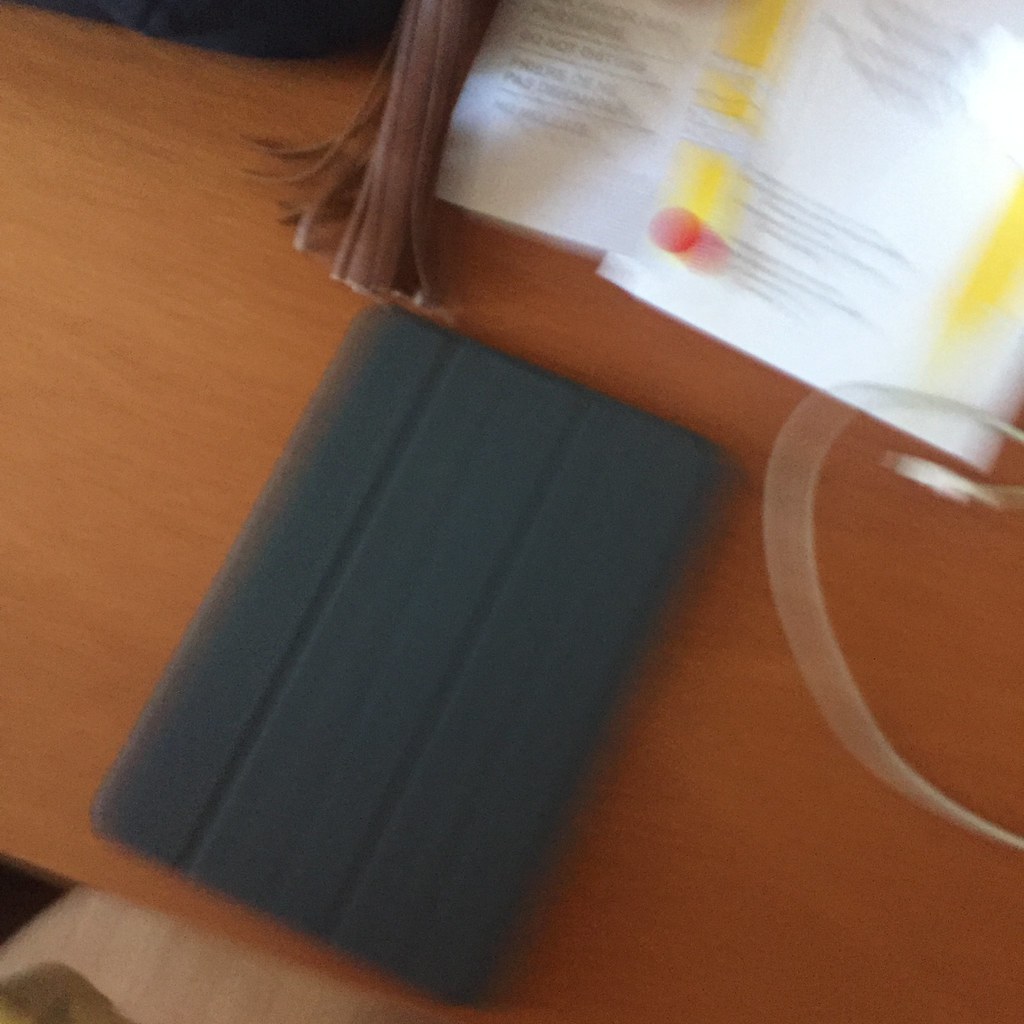This photograph showcases a detailed yet somewhat blurry scene of a workspace. Central to the image is a tablet encased in a dark gray carrying case, segmented into thirds, lying on a reddish wood surface, likely cherry wood. Positioned to the top right of the tablet is an open book, which includes several visible bookmarks. Next to the book lies a brown tassel made of leather or suede. The wooden surface beneath these objects, despite its precise identification as either a desk or table being unclear, clearly exhibits an elegant reddish hue. Additionally, the floor in the background of the room features a light wood texture, adding a contrasting element to the composition.